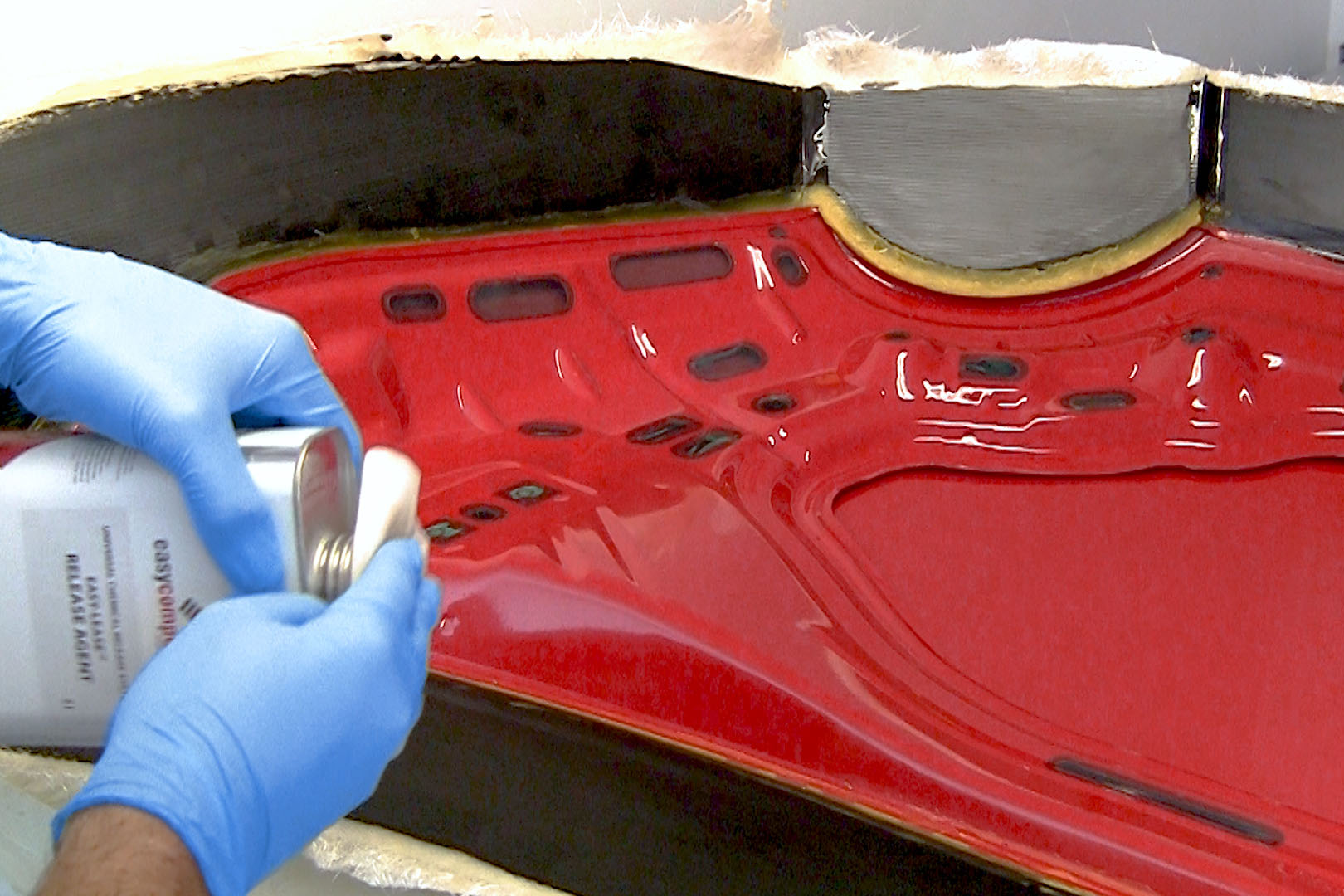The image depicts a pair of hands, covered in blue latex gloves, positioned on the left side of the frame, manipulating a metal canister labeled "EZCOMP" with the additional legible text “release agent.” The man is tilting the canister, allowing a liquid to dispense onto a white tissue. This action seems to be preparing to apply the liquid onto a shiny, red automotive part that dominates the middle to right side of the image. The part, which appears to be either a carbon fiber bonnet or the interior of a car trunk, features black scoping areas, gray structural elements, and various oval cutouts. The automotive surface is intricately curved and has a lacquered finish. In the backdrop, there’s a daylight scene hinted by the remnants of sunlight peeking through some clouds.